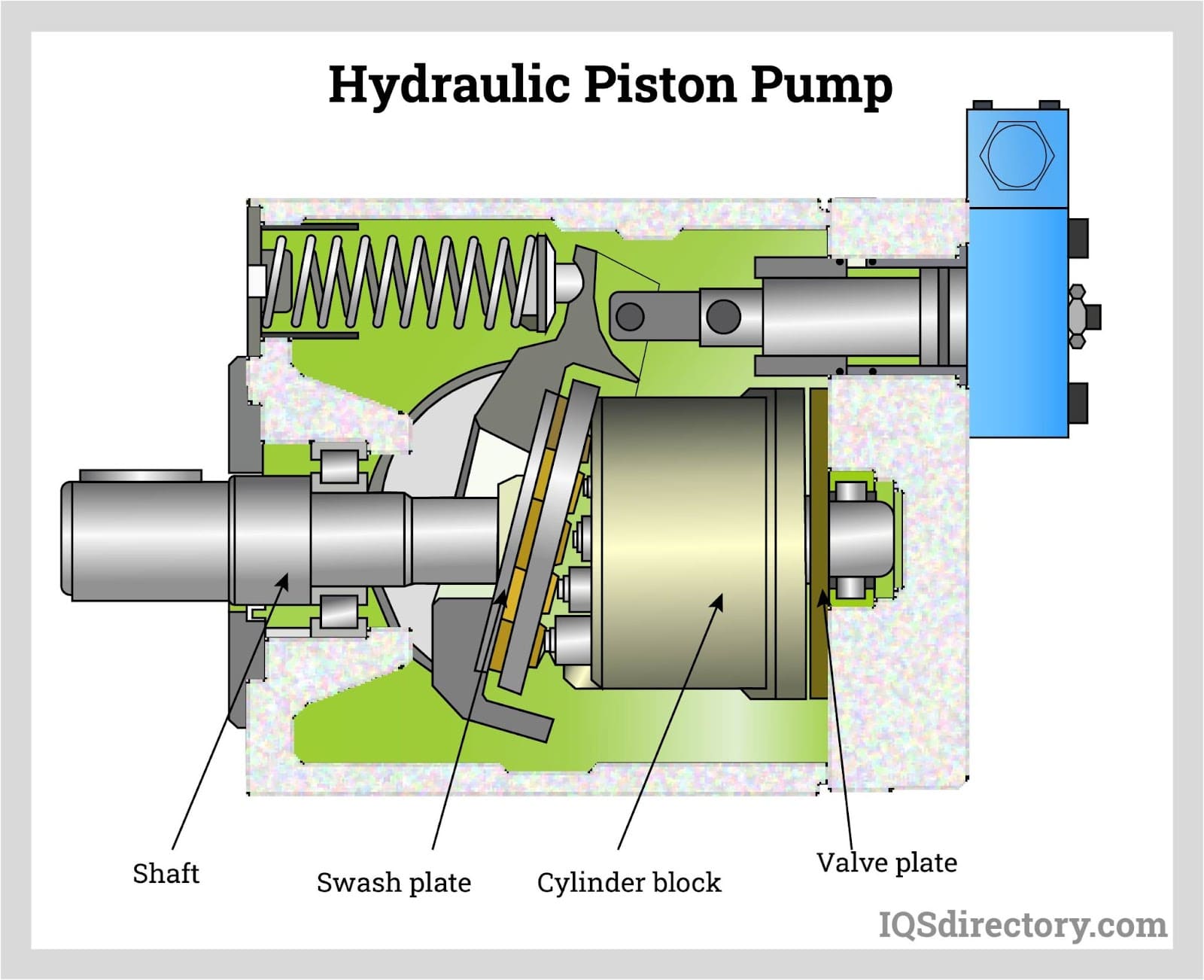The image is a detailed diagram illustrating the internal structure of a hydraulic piston pump in a cross-sectional view. The pump's components are meticulously labeled for clarity. The diagram shows:

1. **Shaft** - a silvery gunmetal shaft that begins the assembly.
2. **Swash Plate** - this is connected to the shaft and is depicted as a swash plate bar.
3. **Cylinder Block** - a tan-colored cylindrical component with multiple smaller cylinders protruding from it.
4. **Valve Plate** - a vertical brown bar situated at the rear of the pump.

The image uses a variety of colors, including gray and green for the metal parts, as well as hints of blue and light gold, adding a vibrant yet technical feel. Some background elements resemble confetti, mimicking the operational motion of the pump. The diagram is sourced from IQSDirectory.com, as noted in the bottom right corner.